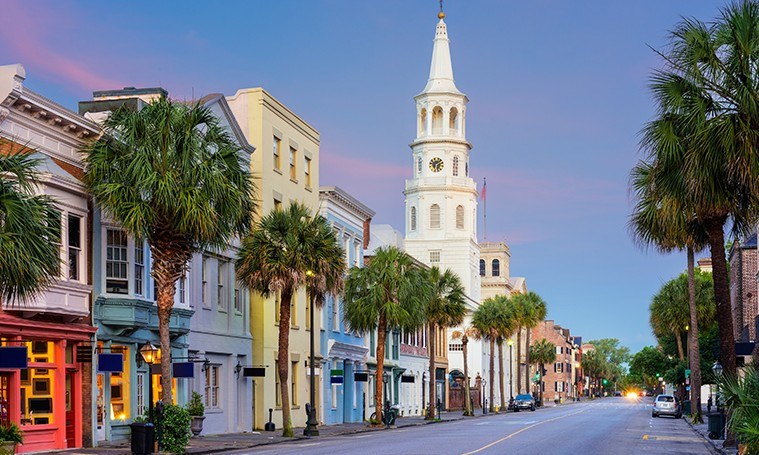The image captures a vibrant main street in a small tropical town as sunset approaches, casting a soft mix of blue and pink hues across the sky. The scene is dominated by a seemingly empty two- or three-lane road with cars parked along both sides and a single car visible in the far background. Both sides of the street are lined with colorful buildings of varying heights, ranging from two to four stories. These buildings are painted in an array of bright colors, including blue, light yellow, purple, red, and turquoise, creating a lively atmosphere. On the left, the buildings stretch from the bottom left to the middle left of the image, while on the right, the road continues into the distance, illuminated by a few bright orange lights at the vanishing point. Halfway down the street stands a prominent white cathedral with a tall steeple, featuring a clock and towering above surrounding structures. Palm trees are evenly spaced along the sidewalks on both sides, adding to the tropical feel. While bicycles and other items are sporadically placed along the way, no people can be seen, giving the impression of a quiet moment in this otherwise lively town center.